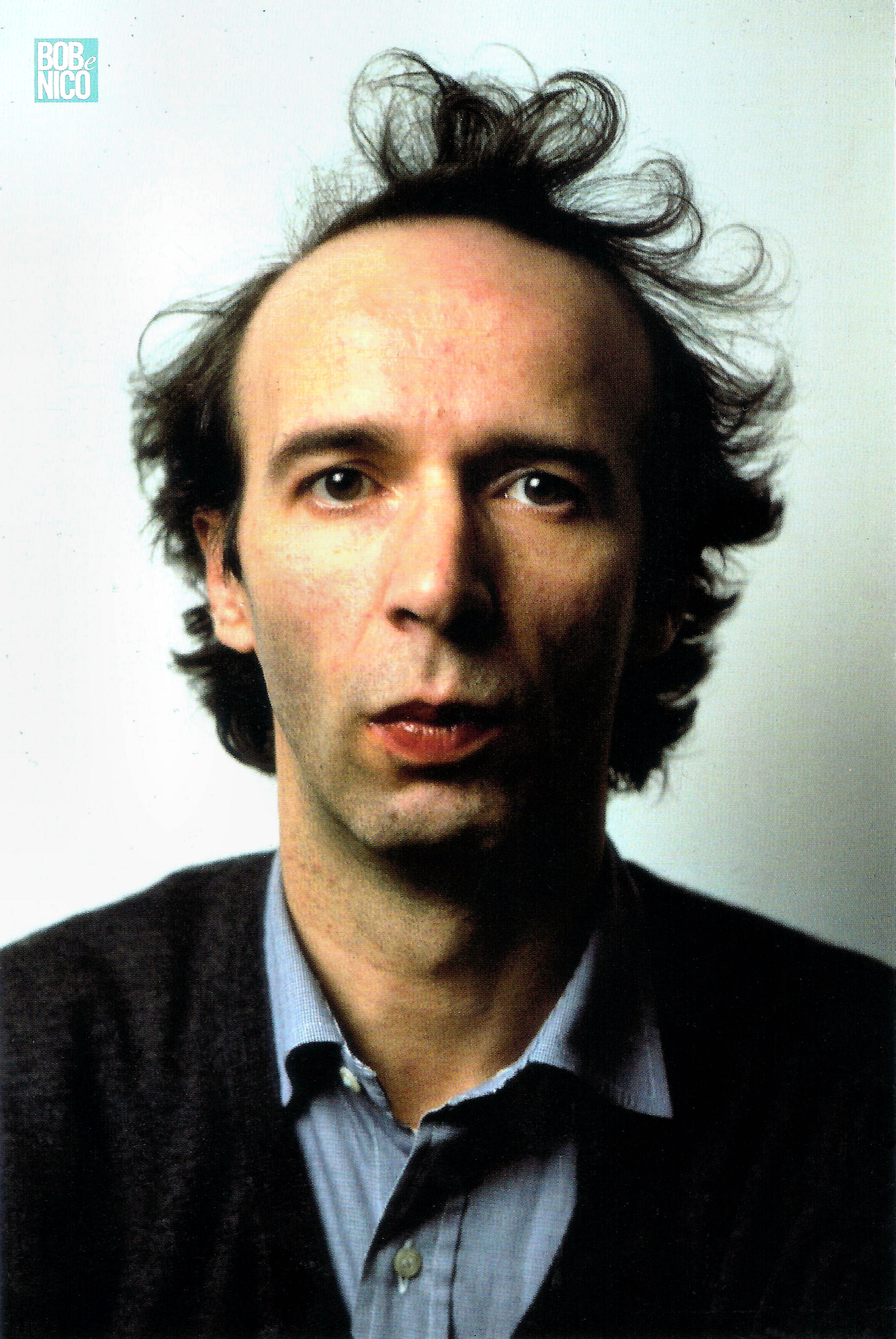This detailed close-up photograph captures a middle-aged man in front of a bluish background that fades from light to medium from left to right. In the upper left-hand corner of the image, there's a blue square with white writing that reads "Bob Nico." The man's head is slightly cut off at the top, revealing his full skull but not all of his hair, which appears wild, short, and unruly, showing signs of balding. He wears a dark, possibly black, v-neck sweater over a light blue button-down collared shirt that peeks out at the neckline. The man's expression is stern with his lips pursed, giving an impression of seriousness or anxiety. His dark brown eyes are clearly visible, along with the slight shadow he casts against the background. He appears to be around 45 to 48 years old and has no facial hair.